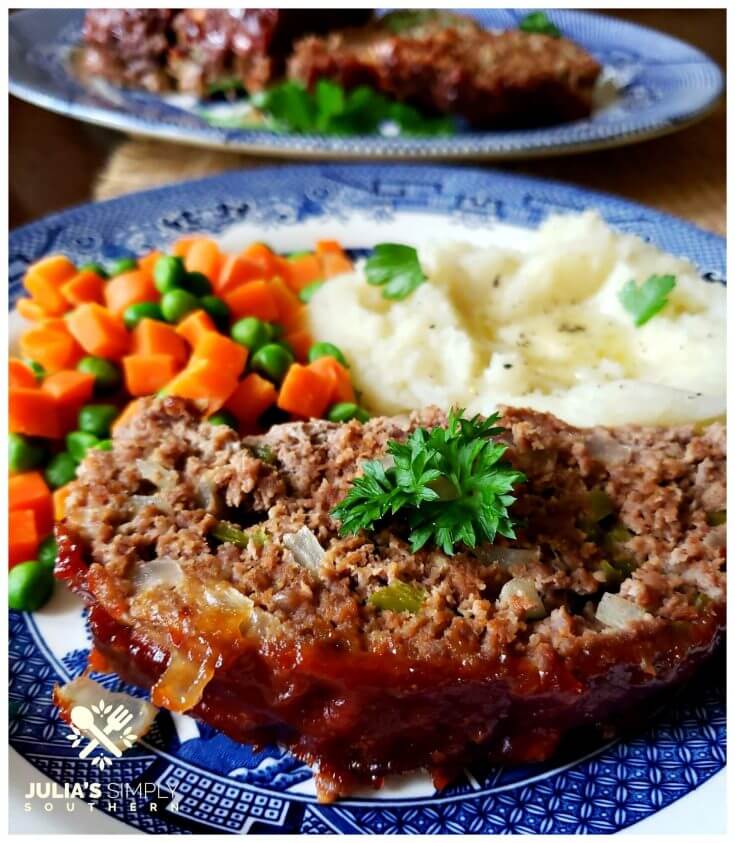This close-up, vertical photograph showcases two blue plates with intricate white, almost medieval, Catholic designs on the edges, placed side by side on a brown wooden table. The plate in the foreground, prominently displayed and in focus, features a slice of meatloaf topped with barbecue sauce, cut and lying on its side. The meatloaf reveals an interior mix with diced onions and bell peppers. Garnished with green parsley, the plate's composition includes a portion of brilliantly colored small diced carrots and peas on the left, and a generous scoop of seasoned mashed potatoes with green flecks on the right. The background plate, slightly blurred, holds three slices of meatloaf topped with celery, void of any additional vegetables. The detailed array of ingredients and the careful presentation create a visually appealing culinary scene.